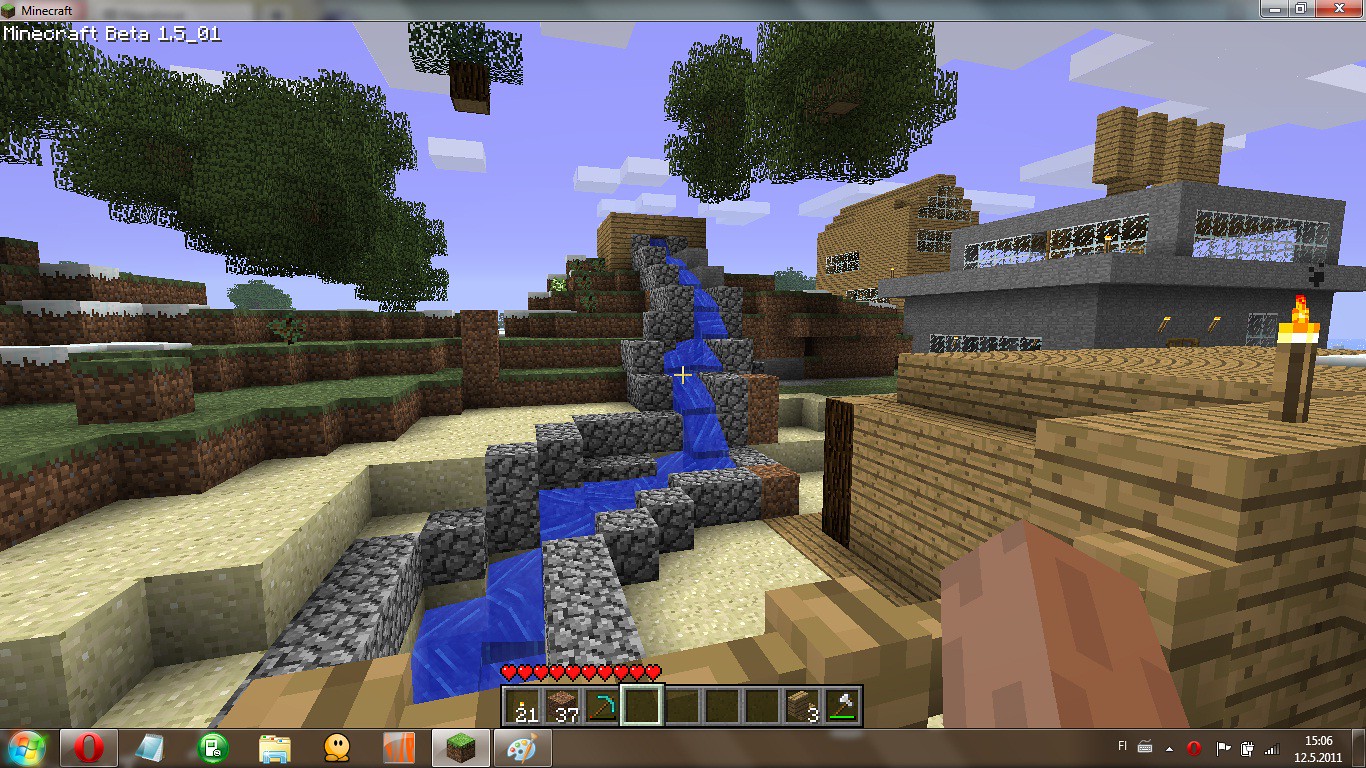The scene is set in a video game world where everything is constructed from blocks. Prominently, water flows down a hill bordered by gray blocks. Adjacent to these gray blocks are tan blocks, with green and brown blocks flanking either side. Floating above are green bushes suspended in the sky, adding a touch of whimsy to the landscape. A torch mounted on a wooden pillar stands to the right, illuminating a two-story stone building. This structure features clear blocks on two sides, presumably windows. Above the stone building, a couple of brown pillars rise, behind which a brown block house with a pointy roof is situated. The source of the water appears to be a large, square, brown structure at the top of the hill.